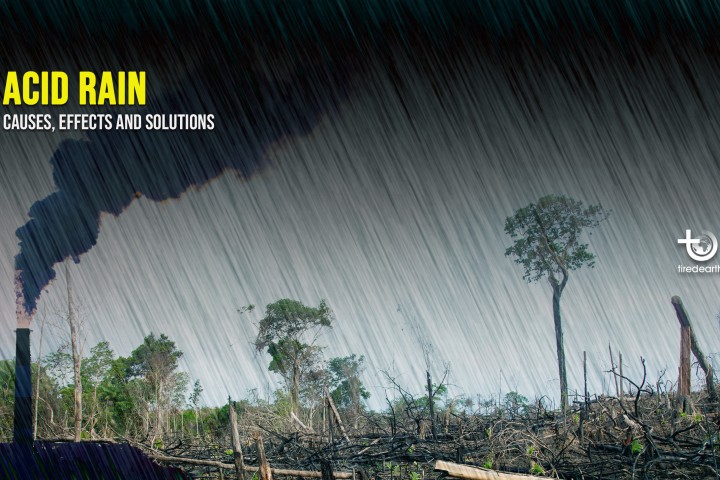This horizontally aligned, borderless photograph vividly depicts the harrowing effects of acid rain on a forest landscape. The upper left-hand corner features bold yellow all-caps text reading "ACID RAIN," with smaller white all-caps text beneath it stating "CAUSES, EFFECTS, and SOLUTIONS." The top portion of the image is solid black, transitioning down to show a smokestack on the left side. This smokestack, attached to a black vehicle in the lower left corner, billows black smoke upwards towards the middle upper side of the image. Diagonal gray lines, symbolizing acid rain, stretch across the scene from this smoke. 

The bleak ground below is littered with sticks, brush, and predominantly dead, leafless branches, although a few trees withstanding the devastation stretch upwards. On the far right edge of the image, the white text "TIRED EARTH" accompanies a logo featuring a 'T' and a globe. The overall scene starkly illustrates the destructive impact of acid rain on the environment, emphasizing the urgency of addressing its causes, effects, and potential solutions.